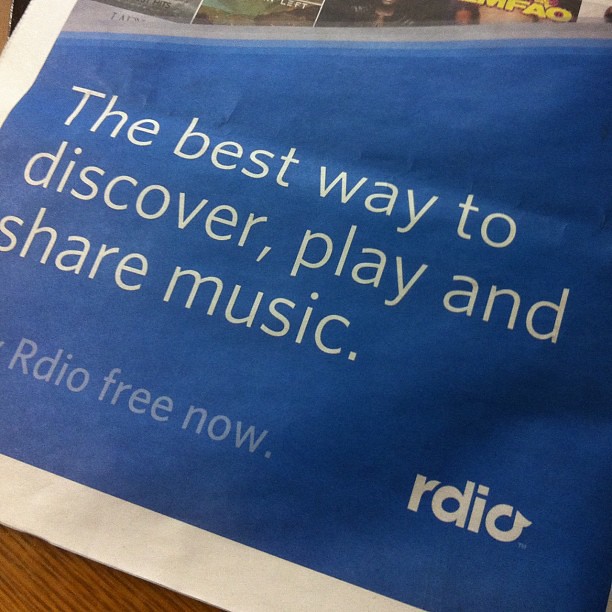The image appears to be a clipped section from a magazine or newspaper, prominently featuring a banner advertisement. The bottom half of the page showcases a rich blue background with an ad text in large white font that reads, "The best way to discover, play, and share music." Beneath this text, in a lighter blue or purple shade, it states, "RDIO, free now." The advert is bordered in white against the blue backdrop, and the lower right corner features the RDIO logo in white. The ad appears to be resting on a wooden surface, with visible wood grain patterns peeking out from the bottom of the image.